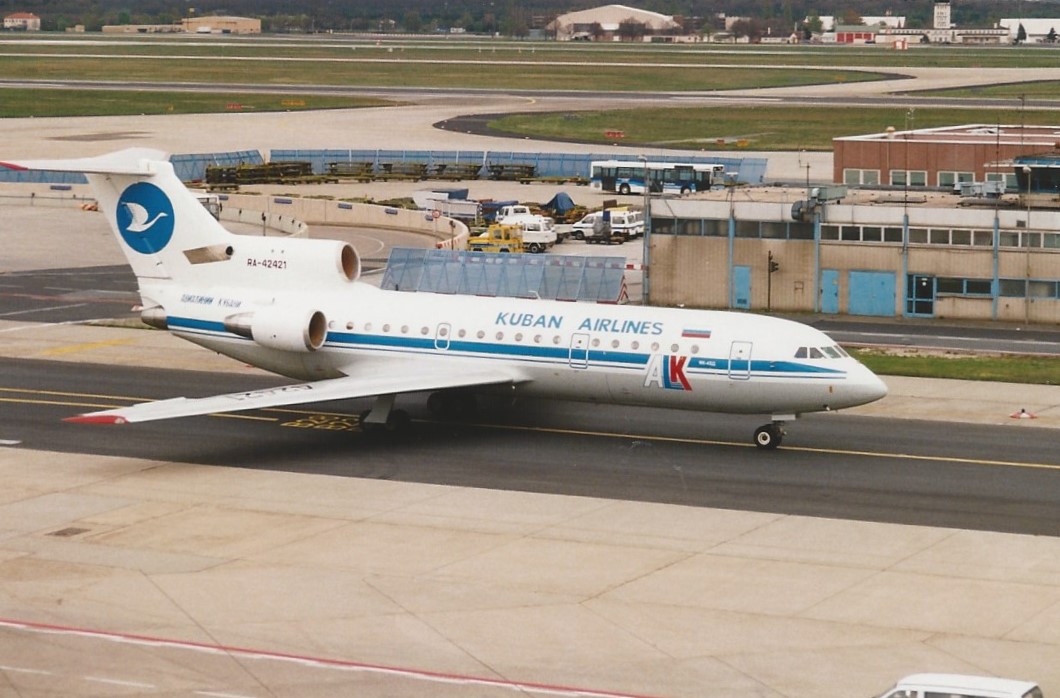The detailed color photograph captures a white airliner positioned on a runway, facing the right side of the image. The airplane prominently displays "Cuban Airlines," spelled as K-U-B-A-N Airlines in blue text, along its fuselage. A distinctive blue stripe runs down the center of the aircraft, accompanied by the initials ALK in white, blue, and red lettering towards the front. The aircraft is marked with the registration number AL-42421. The tail section showcases a logo featuring a white swan flying within a blue circle. The wing of the plane is noteworthy for its red-tipped edge.

In the foreground, there is a concrete pavement area where a small van is visible in the bottom right corner, facing the left. The airplane rests on an asphalt runway marked by a yellow line. Behind the airplane, there is a secondary strip of runway bordered by a grassy area. Further back, several buildings and a shuttle bus can be seen, along with additional work vehicles. In the distant background, a mix of red and large buildings, possibly farm structures, stretches across the horizon.